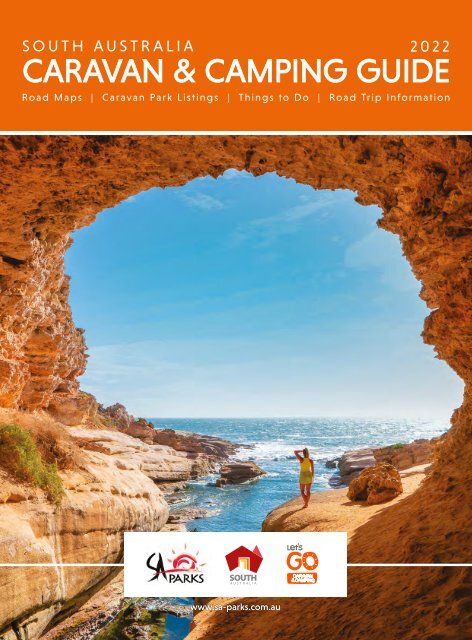The image is the cover of the "South Australia Caravan and Camping Guide 2022." The top portion of the image features a prominent orange bar with white text that reads: "South Australia Caravan and Camping Guide 2022 - Roadmaps, Caravan Park Listings, Things to Do, Road Trip Information."

Below this text, there is a striking vertical rectangular photograph. The photo captures a rugged landscape with a rough-textured, brown rock archway towering over smoother beige rocks. Underneath the arch, a small inlet of water flows through the rocky terrain and extends out into a vast, glistening blue ocean under a sunny sky. High-altitude clouds can be seen in the distance, adding to the scenic beauty.

In the bottom right corner of the photograph, a young woman dressed in yellow stands on one of the smooth rocks, looking out towards the ocean. The sunlight, coming from the upper right, enhances the vividness of the scene.

At the very bottom of the image, there is a white horizontal rectangle with three logos and related text. These logos include SA Parks, a red house icon with the word "South" underneath it, and a logo that says "Let's Go." The website www.sa-parks.com.au is also mentioned, indicating further information and sponsorship details.